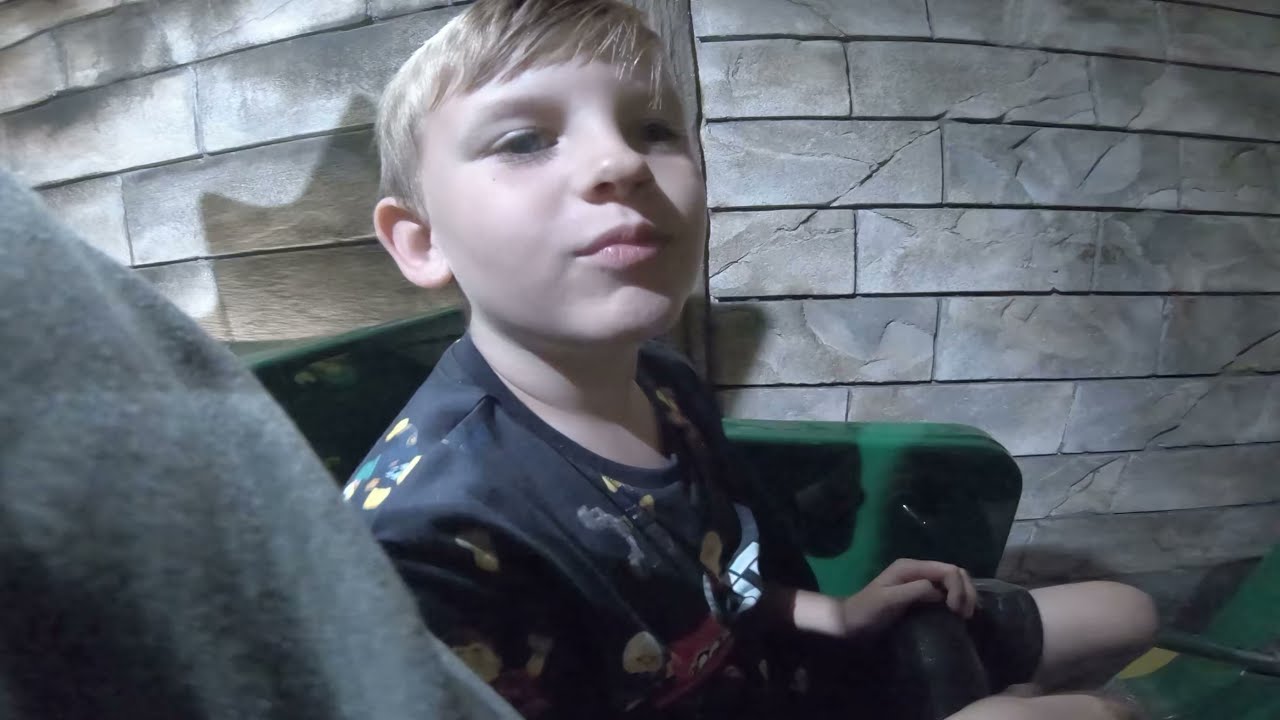The image depicts a young boy, approximately five or six years old, sitting in a green sofa chair. He appears to be indoors, possibly in a house, with an interesting concrete brick wall as the backdrop. The boy, a young Caucasian male with blonde hair, is clad in what looks like pajamas, specifically shorts. Positioned slightly off-center, he's looking towards the camera but with a slight gaze to the right. He's holding something, which could be a pet or a video game controller. The palette of the scene is diverse, featuring colors such as gray, black, dark blue, light blue, yellow, red, tan, green, and various shades of gray. There is another person in the bottom left of the image, mostly cut out, wearing a gray sweater. Additionally, a shadow with spikes, possibly from a statue or furniture, is visible in the background.